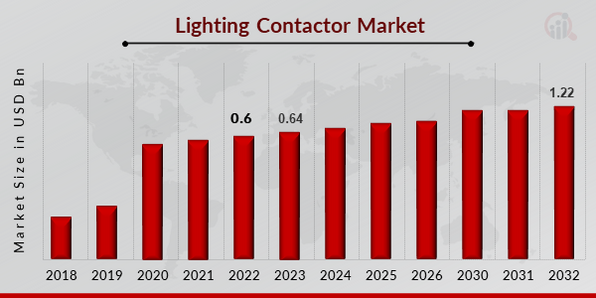The image is a horizontally aligned, rectangular bar graph measuring approximately four inches wide by two inches tall, with a light gray background that subtly features a darker gray map of the US and Europe. At the top, the graph is titled "Lighting Contactor Market," underlined with a black line that has dots at each end. The y-axis is labeled "Market Size in USDBN" in black print, while the x-axis displays years from 2018 to 2032, though it skips 2027 through 2029. Each year is represented by a vertically aligned red bar, with the heights of the bars exhibiting an increasing trend from left to right, starting with the shortest bars in 2018 and 2019, and culminating in the tallest bar in 2032. Specific values are marked: 0.6 for 2022, 0.64 for 2023, and a projected 1.22 for 2032.